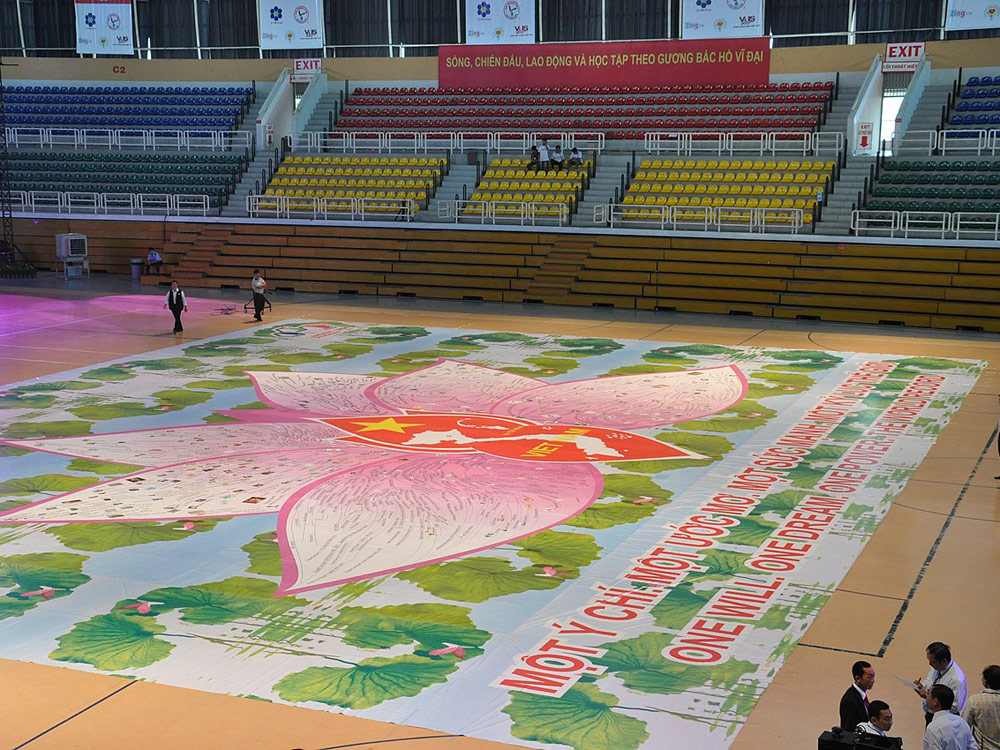The image depicts the interior of a large indoor sports arena or gymnasium in Vietnam, captured in a color photograph in landscape orientation. Dominating the floor is a vast mural featuring a vibrant pink flower with petals radiating from a red center, which showcases the outline of Vietnam in white. Surrounding the mural are multicolored bleachers arranged in sections of blue, green, red, yellow, and black seats, with some brown wooden bleachers court-side. Further up in the stands, a red and white exit sign is visible. 

An array of posters and banners, including one with red text in Vietnamese and another proclaiming "One will one dream," embellish the setting. In the bottom right corner, a group of people, dressed in white shirts and suits, are engaged in conversation, suggesting the presence of officials or judges. The gymnasium is illuminated by a pink light, adding to the vibrant atmosphere of the scene.